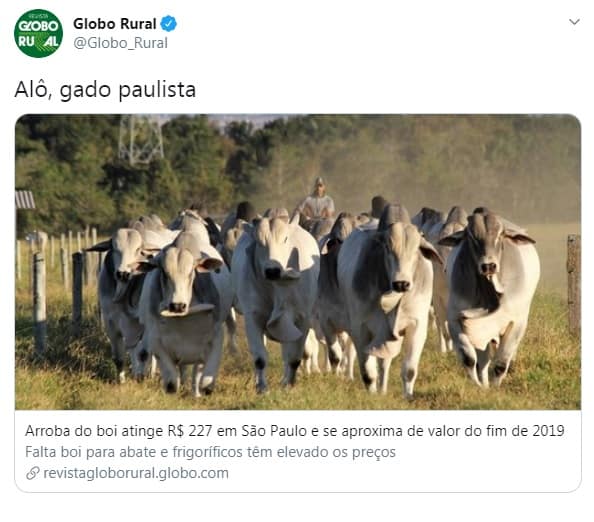The image is a screenshot from a Global Rule tweet, identifiable by their verified blue check mark. It features an outdoor scene with a herd of large, white cattle being herded by a farmer on horseback with a gray shirt. The cattle are moving towards the camera across a grassy field, creating a cloud of brown dust. The background is lined with a row of trees, and there is a wooden fence on the left side of the field. The Global Rule logo, featuring a green symbol with white lettering, is at the top of the tweet, which contains an article in Portuguese. The article's title is "Elogado Paulista," and further down, it reads, "Arroba do Boi atinge R$227M em São Paulo e se aproxima de valor do final de 2019. Falta boi para abate e frigoríficos, tem elevado os preços." The tweet links to "revistagloborural.globo.com," indicating this news article discusses the high value and scarcity of cattle for slaughter, contributing to rising prices.